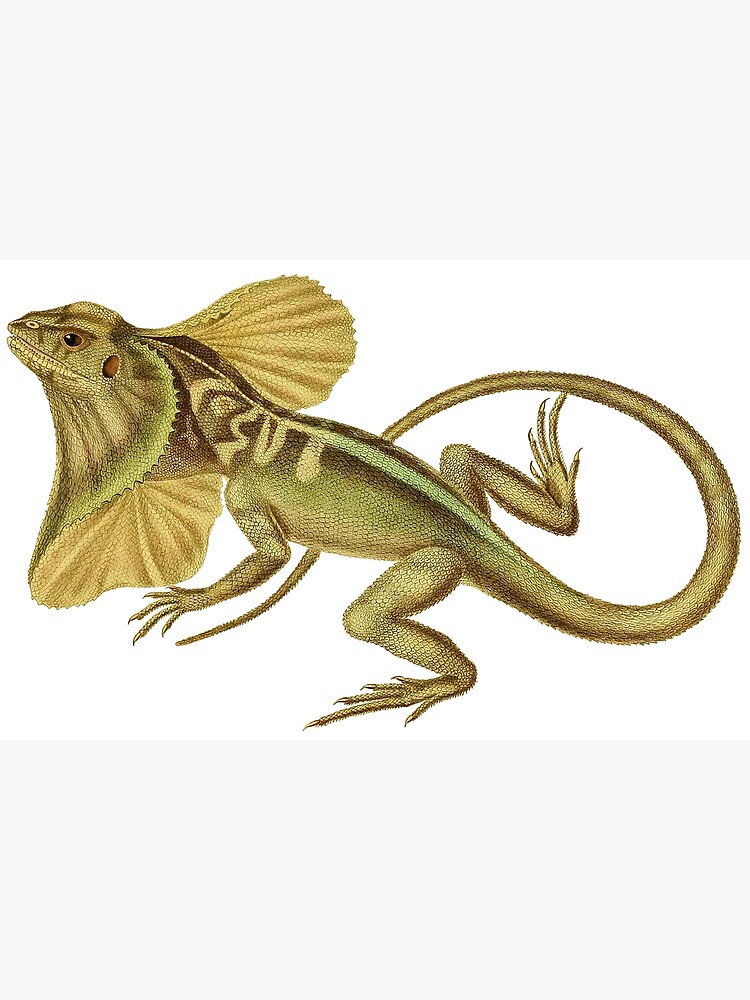A detailed drawing depicts a green lizard with a notable hood that is currently fanned out, giving the creature a distinctive, expanded neck appearance. The lizard resembles a newt or salamander in body structure and has five clawed fingers on each foot. The lizard's skin is a rich green color with lighter green and yellow-green markings, especially prominent on the underside of the hood. It features small black eyes and a tiny nostril hole. The creature has small, pointy teeth visible in its slightly open mouth. Its elongated tail is curled underneath its body, and the lizard stands against a stark white background. The creature's neck is notably elongated, and its back sports darker green and black patterning with a central light green stripe and several lines extending from it. The sides of the lizard are lighter in green, transitioning to a yellow hue on its underbelly and legs.